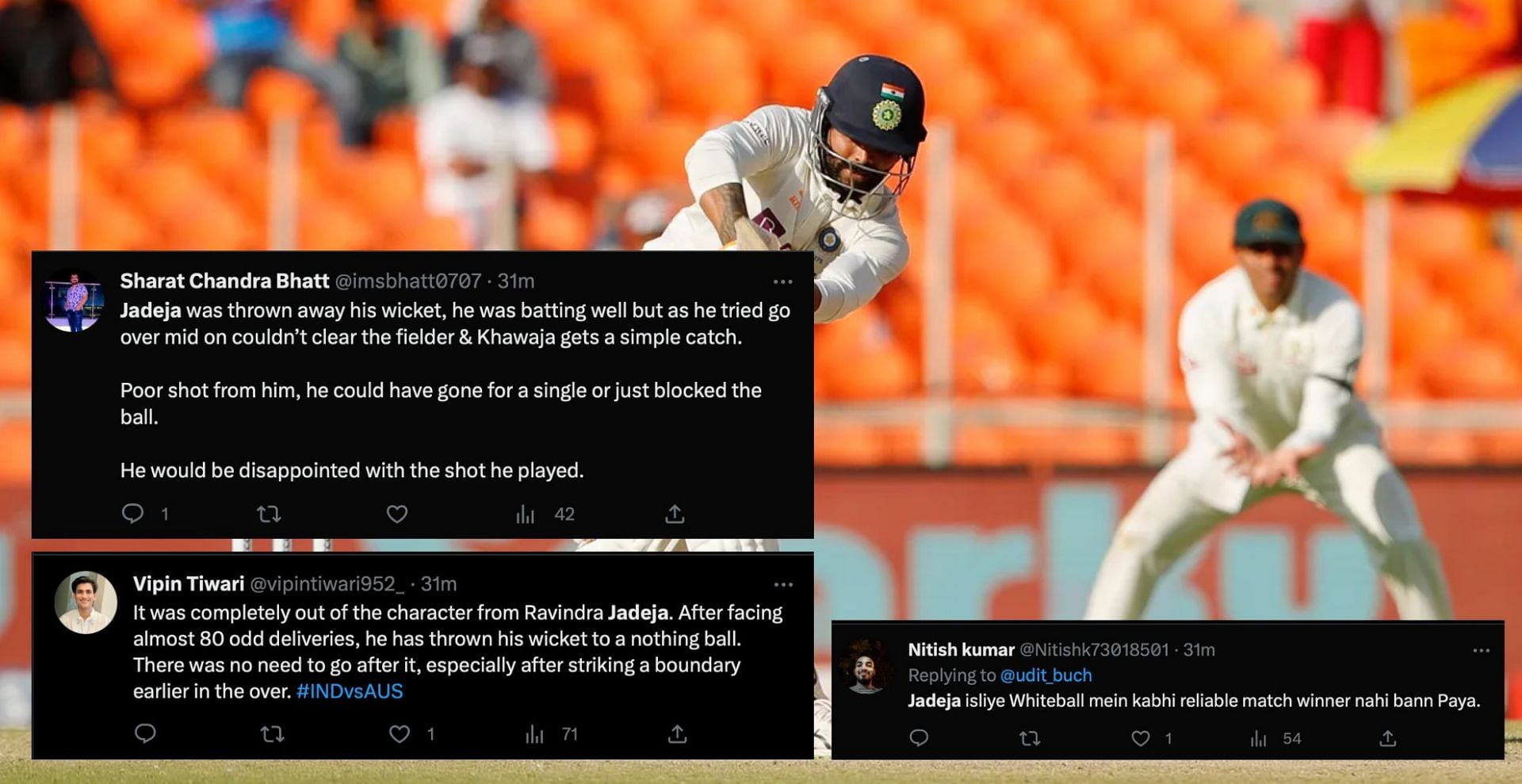The image captures a high-quality, professionally taken photograph at a baseball game, focusing centrally on a player who appears to be swinging a bat. The player's face is somewhat obscured by three superimposed screenshots of tweets, making it difficult to see exactly what he's doing with the bat. He’s wearing a navy blue helmet and a white long-sleeve shirt. The catcher behind him, also dressed in similar white clothing, is squatting with his hands outstretched, poised to catch the ball, and wears a dark navy blue or black baseball cap. The background reveals rows of orange seats in a stadium, occupied by a few spectators. 

Superimposed tweets add a layer of narrative, discussing a cricket match involving Ravindra Jadeja, which creates an interesting juxtaposition against the baseball scene. The tweets critique Jadeja's performance, mentioning how he threw away his wicket by attempting a risky shot that was easily caught. They express disappointment over his poor decision-making despite his earlier good form, contrasting sharply with the depicted baseball image.